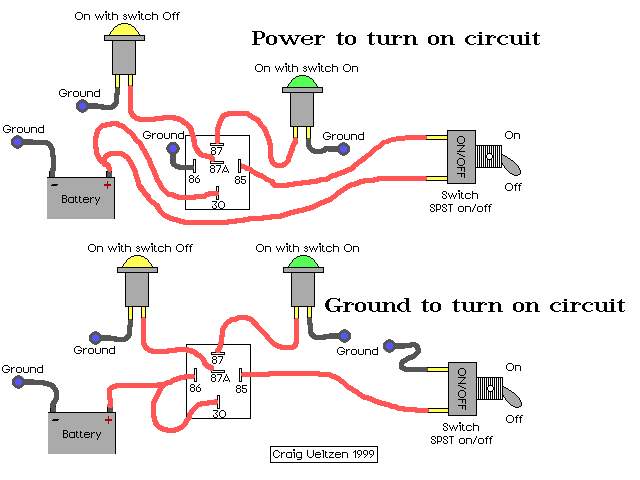The image depicts two detailed electronic circuit diagrams set against a white background. Both diagrams run horizontally from left to right and are primarily gray with significant red wiring. The upper diagram features a black heading stating "Power to Turn On Circuit," while the lower diagram states "Ground to Turn On Circuit." Each diagram shows red wiring originating from a ground battery, which connects to multiple on and off switches, indicating control points in the circuitry. The upper diagram includes two on/off switches in sequence before a final on/off switch at the end.

The lower diagram mirrors the upper one but features an indicator light in the middle. Both diagrams incorporate a numbered circuit board labeled 87, 87a, 85, 86, and 30, illustrating consistent connection points and control elements across both designs. Additionally, the signature "Greg Litson 1999" is visible below these diagrams, suggesting authorship and date of creation.